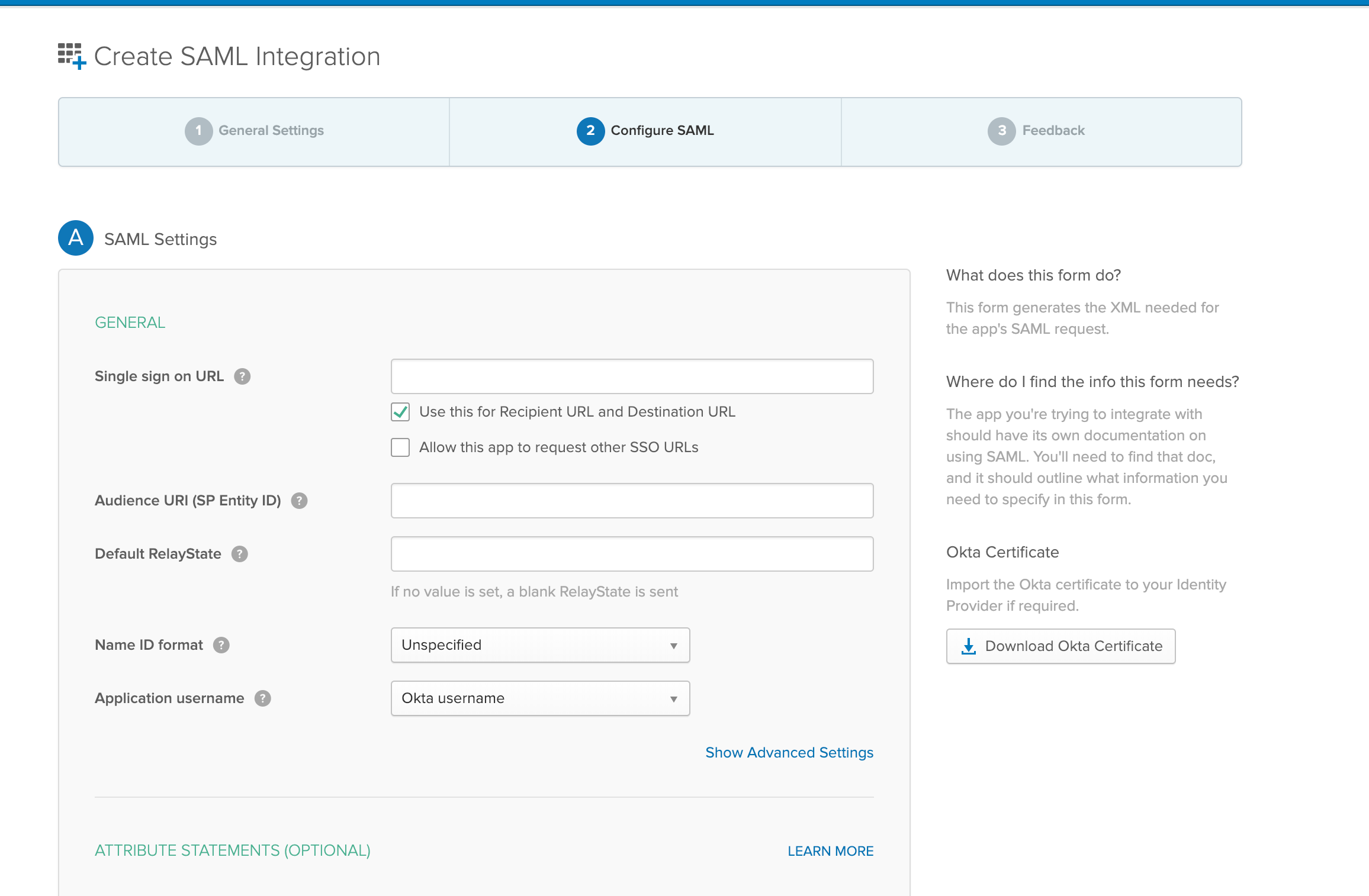In this detailed depiction of the screenshot taken from an online interface, the image is set against a stark white background. At the top, there is a prominent blue horizontal border running from left to right. Within the interface, against this solid white backdrop, there are several blue forms and boxes denoting different segments of the screen. 

In the upper left corner, the text "Create SAML Integration" is displayed in blue. Below this heading, three distinctly outlined options are set against a light blue background - "General Settings," "Configure SAML," and "Feedback" - displayed from left to right. The "Configure SAML" option is highlighted and expanded below, providing further details.

To the left, there's a blue circle containing the letter "A," indicative of the section's focus. To its right, the title "SAML Settings" is prominently displayed. Below this title, a blue box contains the word "General" in blue text.

Proceeding downward, a form is presented with several essential fields, beginning with "Single Sign-On URL" followed by an empty box to its right for input. A checkbox below this box signifies its option, tagged as "Use this for Recipient URL and Destination URL," and it is already checked off.

Further down, the form continues with "Audience URI (SP Entity ID)" and "Name ID Format" which includes a dropdown box currently showing "Unspecified." Finally, towards the bottom, the field "Application Username" is listed, completing this thorough setup for configuring SAML integration.